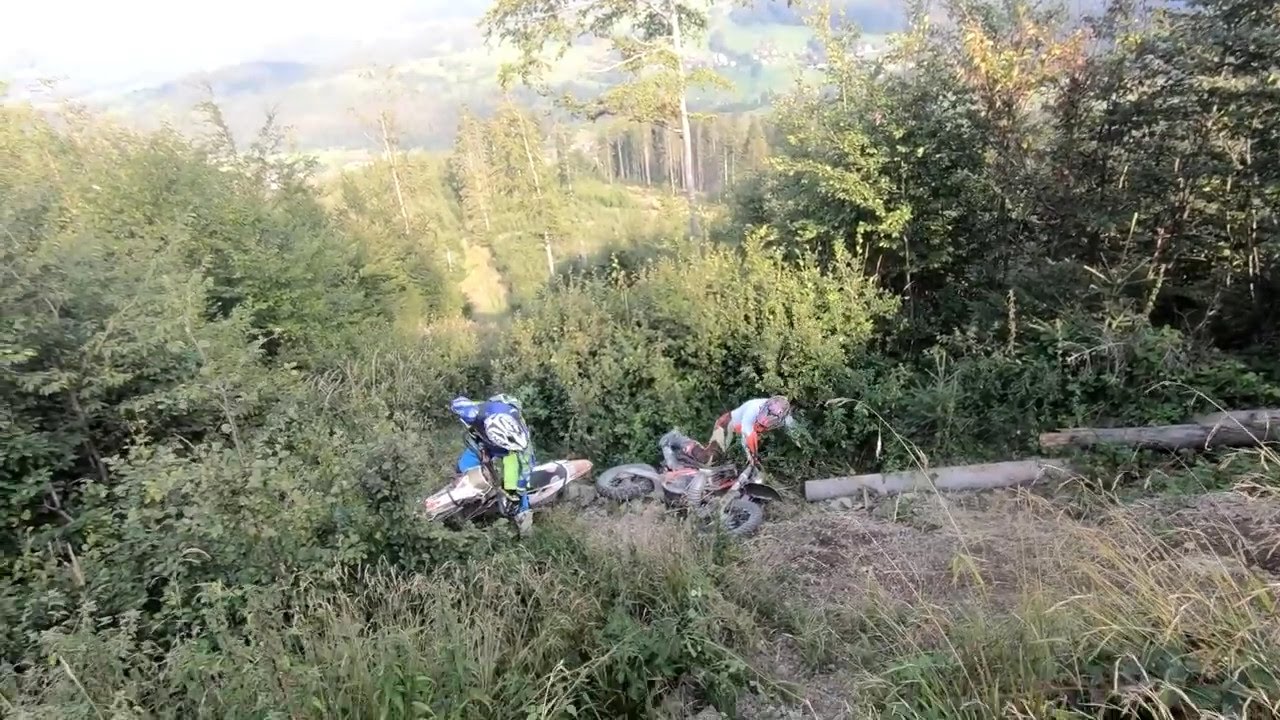This photograph captures a scenic valley view taken from a hilltop. The area is very wooded, with a mix of lush green and brown trees and plants indicating some dryness. The foreground features two bikers with their motorcycles, each wearing helmets and distinct outfits—one biker in a red and white uniform and the other in a blue uniform. The biker in red and white appears to be on his bike, while the one in blue is on the ground near his bike, suggesting a possible fall or minor crash. The landscape is rugged and overgrown, with fallen logs and thick vegetation. The image portrays an expansive view with a cloudy sky, a hint of blue, and a hazy backdrop that includes a dense forest filling the valley, as well as distant mountains. The scene is indicative of a challenging yet picturesque outdoor adventure.